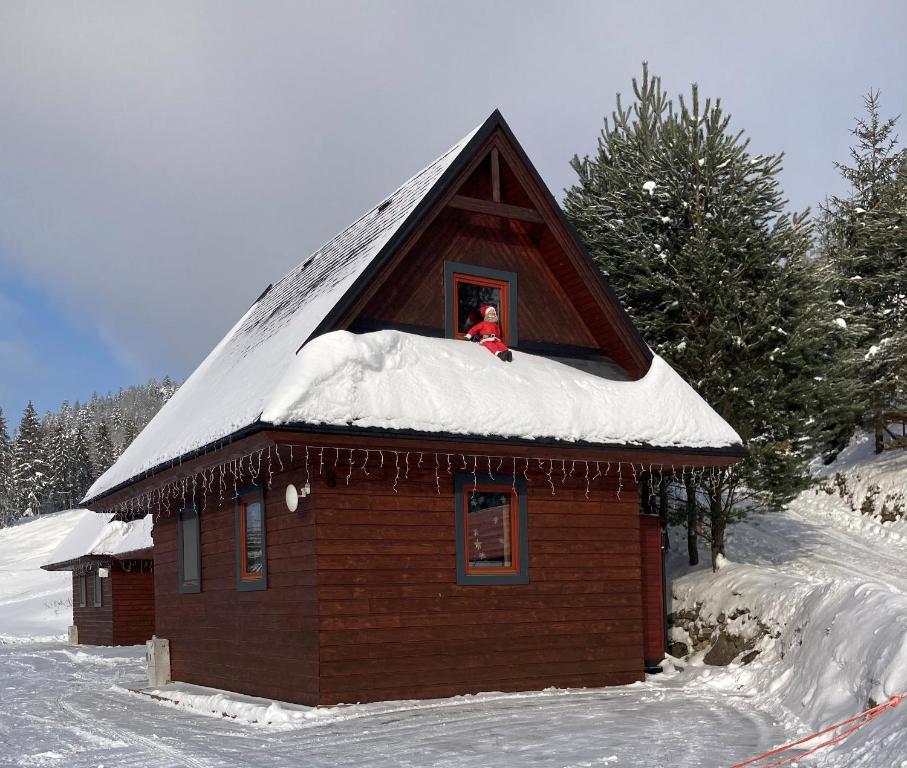The image depicts an exterior shot of a large, A-framed wooden cabin. The cabin, made of wooden planks with distinct blue and red-framed windows, stands prominently in a thickly snow-covered landscape. The snow on the ground and roof emphasizes a wintry atmosphere, while strings of Christmas lights drape from the sides of the roof add a festive touch. The cabin features three lower-level windows and an attic window, in front of which sits a Santa Claus doll nestled in the snow. To the right, a snow-covered path ascends a hill dotted with multiple pine trees. In the background, a portion of an outbuilding is visible behind the cabin, also surrounded by trees with scant snow. The sky above is primarily gray with patches of light blue, completing this serene winter scene.